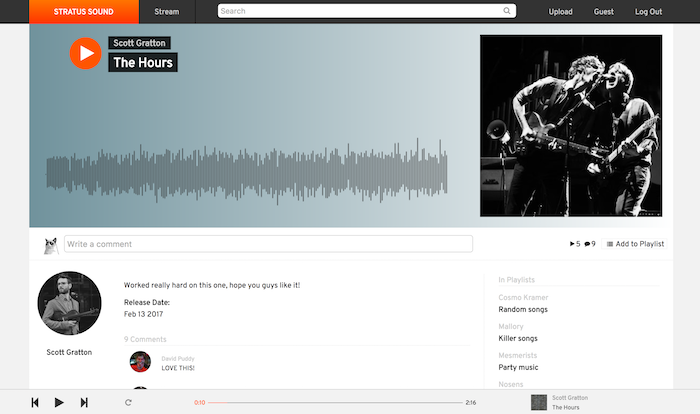This image shows a page from the SoundCloud website. In the upper left corner, there is an orange button labeled "Stratus Sound." The top toolbar is colored dark gray and contains several elements: a button for "Stream," a central search box, and links for "Upload," "Guest," and "Logout" on the right.

Central to the webpage is the SoundCloud audio player, recognizable by its orange play button with a white arrow in the center. Currently loaded in the player is "The Hours" by Scott Gratton. To the right of the player is a black and white photograph of Scott Gratton performing on stage with another musician. Both artists are playing guitars and singing into a shared microphone.

Below the audio player, there is a message from Scott Gratton that reads, "Worked really hard on this one, hope you guys like it. Release date: February 13, 2017," accompanied by Scott Gratton's profile image. Below this message, users have left comments, with the first one stating, "Love this."

On the right side of the page, there are links to additional categories of music such as "Random Songs," "Killer Songs," and "Party Music."